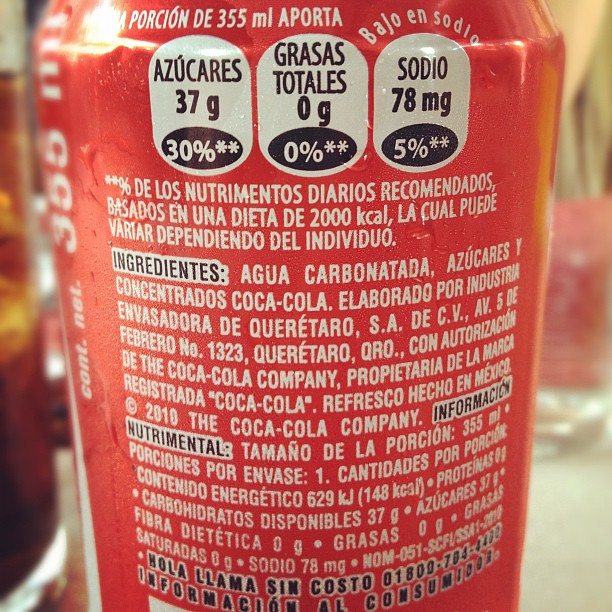This image features the back of a red can of Coca-Cola, labeled entirely in Spanish. The can, presumably a 355 ml serving, displays nutritional information within white ovals. It mentions 37 grams of sugar (30% daily value), 0 grams of total fat (0% daily value), and 78 milligrams of sodium (5% daily value). Below these figures, the ingredients list includes "agua carbonatada" (carbonated water) and "azucares" (sugars). Additional text includes "nutrimenta" and "tomates de la porcion." The bottom of the can displays "hola llama sin costo." This product appears to be part of the Coca-Cola lineup, indicated by a copyright mark and "Hecho en Mexico" (Made in Mexico), with a 2010 copyright date. The can is placed on a table, with the focus primarily on its detailed label.